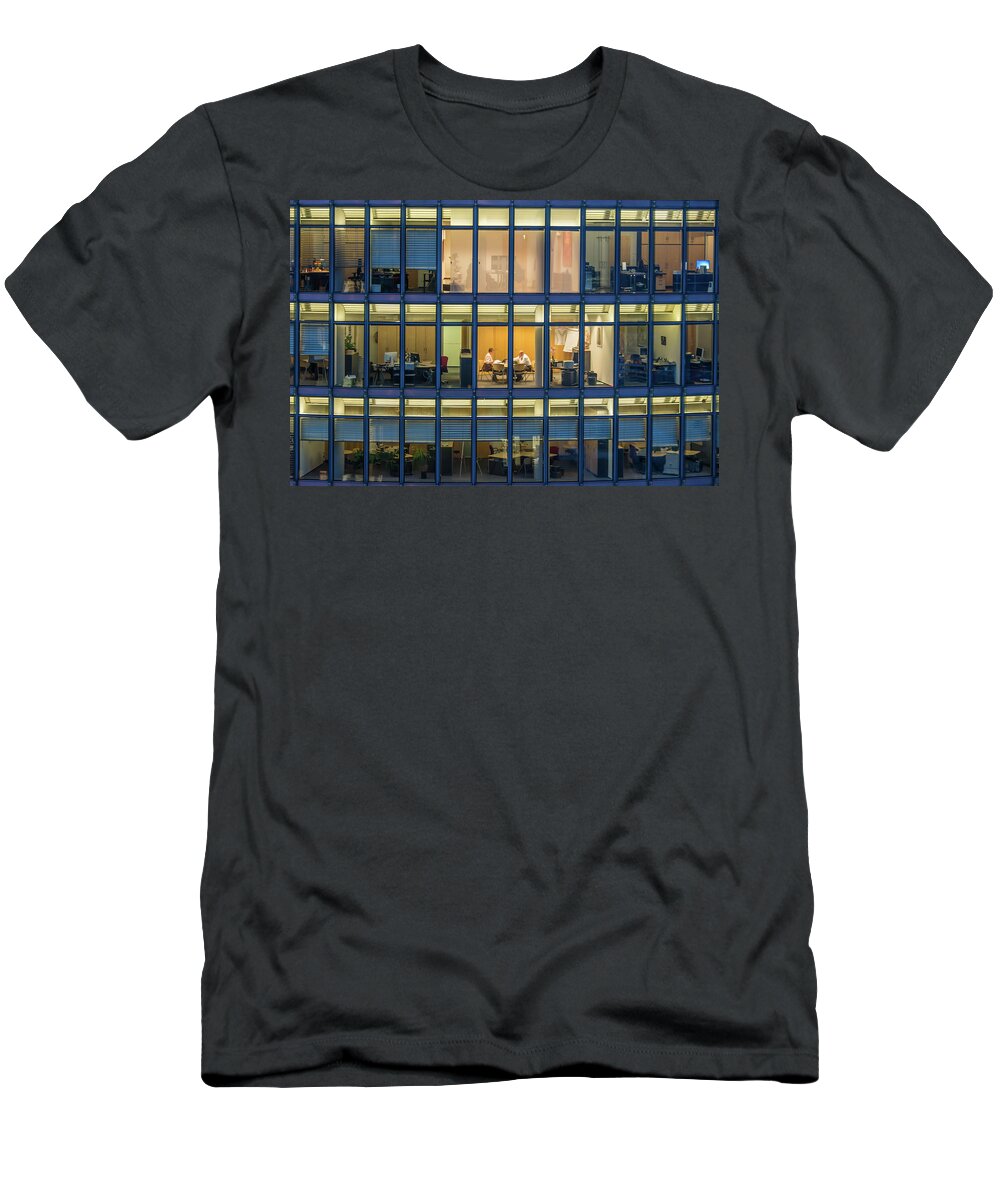This image features a black, short-sleeve crew neck t-shirt laid out flat against a plain white background. The t-shirt showcases a large, detailed image prominently displayed, covering about half of the front and extending almost to the neckline. The image depicts the exterior of a three-story office building with a significant number of windows arranged in three columns and three horizontal rows. Through the windows, various office scenes are visible. Several desks with office equipment are scattered throughout, and some windows have their blinds partially pulled down. The bottom row of windows features desks with the blinds pulled down about a third of the way. The middle row shows more desks, with visible interactions including two men having a meeting. The top row contains additional office equipment and desks, with some blinds partially lowered. The dynamic nature of the scenes, varying from dimly lit spaces to well-lit areas shining with lamps, adds depth and interest to the design on the t-shirt.